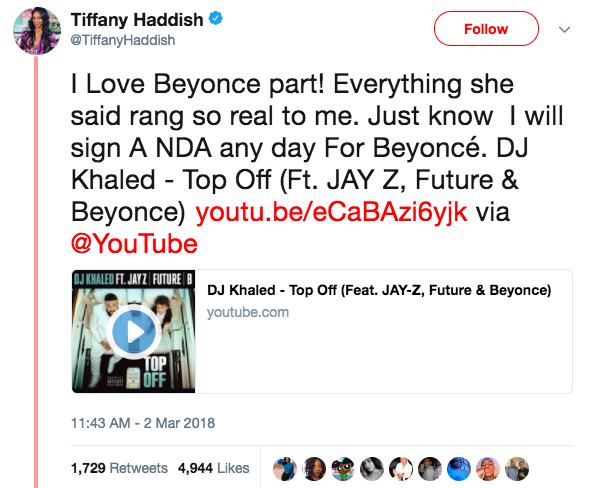On this page, we see a Twitter post by Tiffany Haddish, denoted by her verified handle "@TiffanyHaddish." The tweet, made on March 2, 2018, at 11:43 AM, reads: "I love Beyoncé's parts. Everything she said rang so real to me. Just know I will sign a non-disclosure agreement any day for Beyoncé." Tiffany is referring to Beyoncé's contribution to the song "Top Off" by DJ Khaled, which also features artists Jay-Z and Future. A thumbnail preview of the music video on YouTube is visible within the post. The tweet has garnered significant attention, with 1,729 retweets and 4,944 likes.